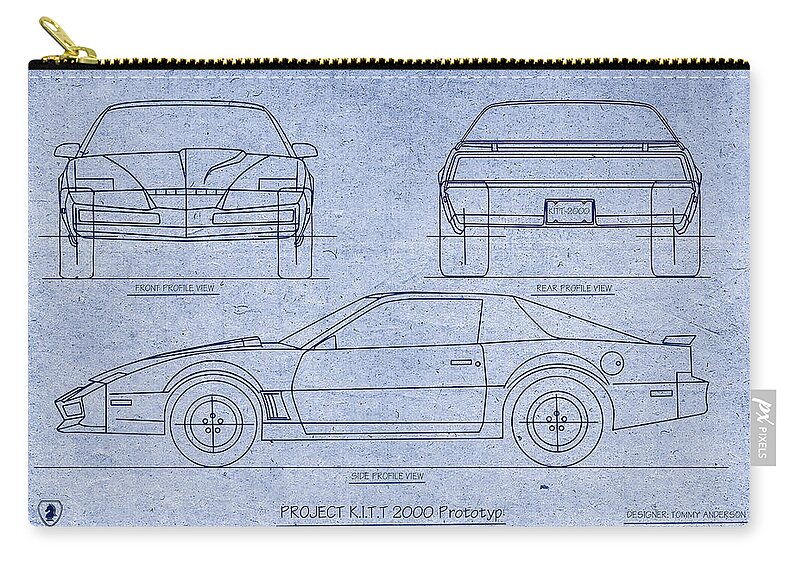The image depicts a rectangular, light blue zippered pouch made of a possibly sturdy fabric or plastic material. The pouch features a prominent brass zipper along the top, secured with white stitching. Across its surface, there is a detailed black line drawing showcasing the schematic views of a sporty car named the "Project KITT 2000 Prototype." The design includes three perspectives: a large side profile view spanning the width of the pouch, a front profile view in the upper left corner, and a rear profile view featuring a license plate marked with "2000" in the upper right corner. Beneath these images, the text "Project K.I.T.T. 2000 Prototype" is underlined and prominently displayed, with the attribution to designer Tommy Anderson. Additional elements include a small tag on the right side labeled "PX Pixels" and a barely discernible logo in the bottom left corner, resembling a seahorse or possibly a chess knight symbol within an inverted triangle. The overall design evokes a blueprint aesthetic, rendering the sporty, Corvette-like vehicle in a technical and modern style.